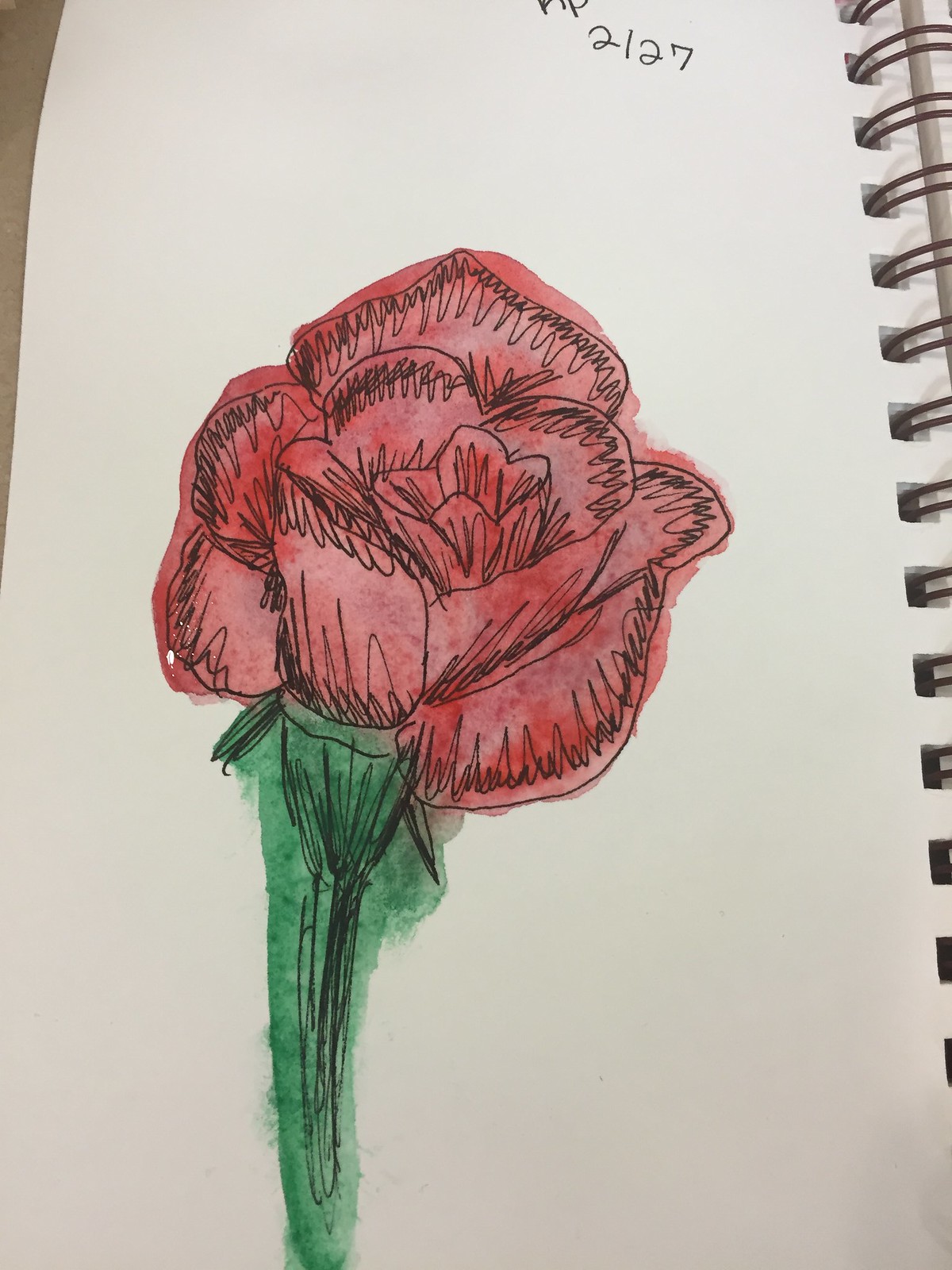In the center of the left page of a spiral-bound sketchbook, a red rose is meticulously illustrated with pen and watercolor. The spiral binding, crafted from black metal wire, is visible on the right side, securing all the pages together. At the top of the page, the faint bottoms of two letters can be discerned, with "2-27" clearly written underneath. The rosebud, tightly closed and just beginning to open, is painted in varying shades of red, accented with black pen details that make the petals' edges pop. Black wavy lines add depth around the petals. The stem is a combination of black ink and green watercolor, creating a nuanced effect with some paint extending beyond the stem’s outline. The overall depiction is both beautiful and intricate, capturing the delicate nature of the flower through careful shading and vibrant color.